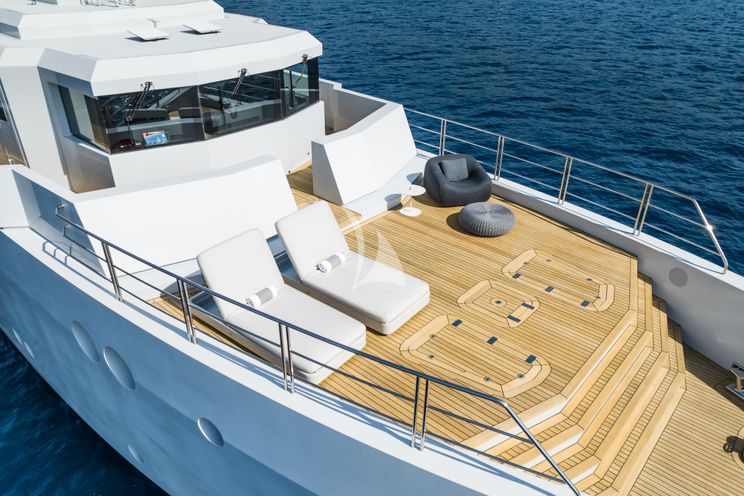The image captures a high-angle view of a computer-generated luxury yacht, possibly AI-generated, showcasing meticulous detail and sophistication. The yacht floats on dark blue, moderately rough water, highlighting the vessel's gleaming white hull adorned with portholes. The deck is constructed of blonde wood and features three steps leading down to a lower level. Two white chaise lounges, each with what appears to be a pillow or towel, are strategically positioned for relaxation. Adjacent to these lounges is a gray easy chair paired with an ottoman, accompanied by a small white table and a little gray circular stand. To the right, a dark beanbag-like chair adds a touch of casual comfort. The deck is surrounded by silver-white railings, ensuring safety. Toward the interior, the bridge area is visible with its sleek black windows and white superstructure, housing a computer or control system that's operational. The yacht's three windshields, equipped with top-down wipers, emphasize its readiness for navigation. Notably absent from this serene and luxurious scene are any people, enhancing the pristine and untouched atmosphere of the yacht on the serene water.